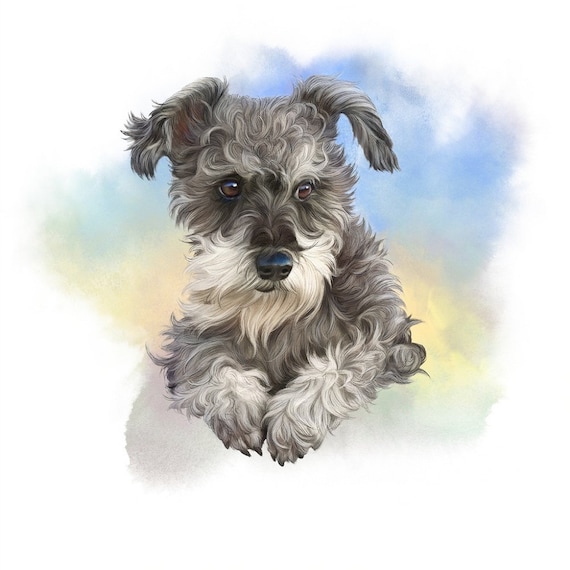This image is a detailed painting of a schnauzer dog, prominently centered in the frame. The schnauzer's curly fur is primarily gray and white, with distinguishing features such as long fur around its mouth, a black nose, and expressive brown eyes. Its front legs, colored a slightly dirty off-white, are extended out front with paws touching each other, giving the impression of the dog lying down. The dog appears to be gazing towards the bottom right corner of the image.

The background is a dreamy mix of blue, yellow, and gray hues, creating an ethereal atmosphere. This misty, cloud-like backdrop combined with a blue sky and touches of gold gives the dog a floating, heavenly appearance, as if it were surrounded by a tranquil and serene aura. The image does not feature any text, maintaining a pure focus on the beautifully rendered portrait of the dog.